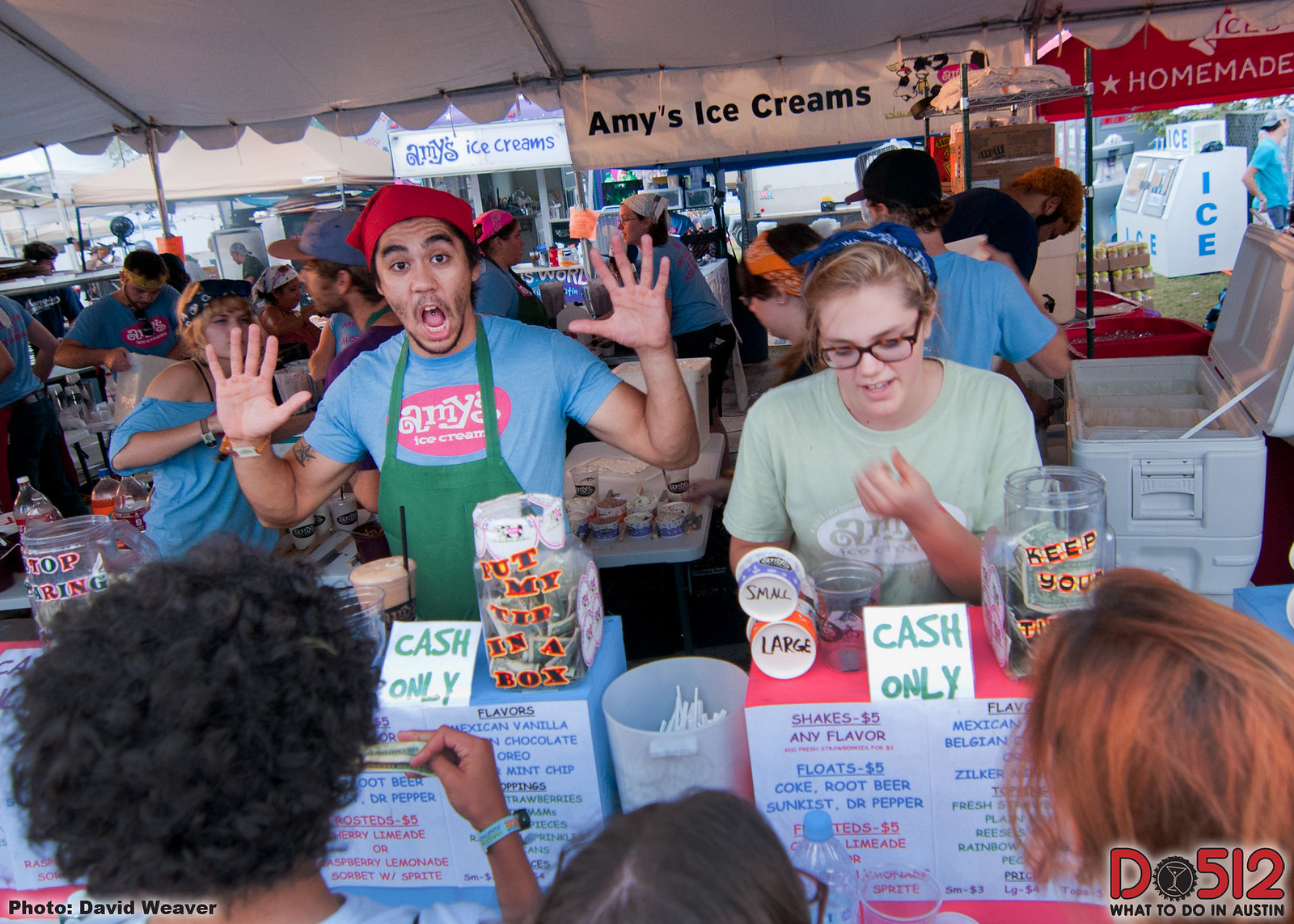At an outdoor market event, two people under a tent are serving as vendors for Amy's Ice Creams, which only accepts cash. A man, standing at the forefront, is wearing a blue "Emmys" T-shirt, a green apron, and a red head covering. He has his hands raised and his mouth open, possibly engaging with customers. To his right is a woman with glasses, wearing a green T-shirt and a blue hair covering. Both are positioned in front of signs listing items such as shakes ($5, any flavor) and floats ($5, available in Coke, root beer, Sunkist, and Dr. Pepper).

In front of the vendors, a person with curly hair, shown from behind, holds money, indicating they are ready to make a purchase. Other signs around their booth also display "cash only" notices. Additional containers marked "Small" and "Large" can be seen. Behind the vendors, several other booths and clusters of people are visible, adding to the lively ambiance of the market scene.